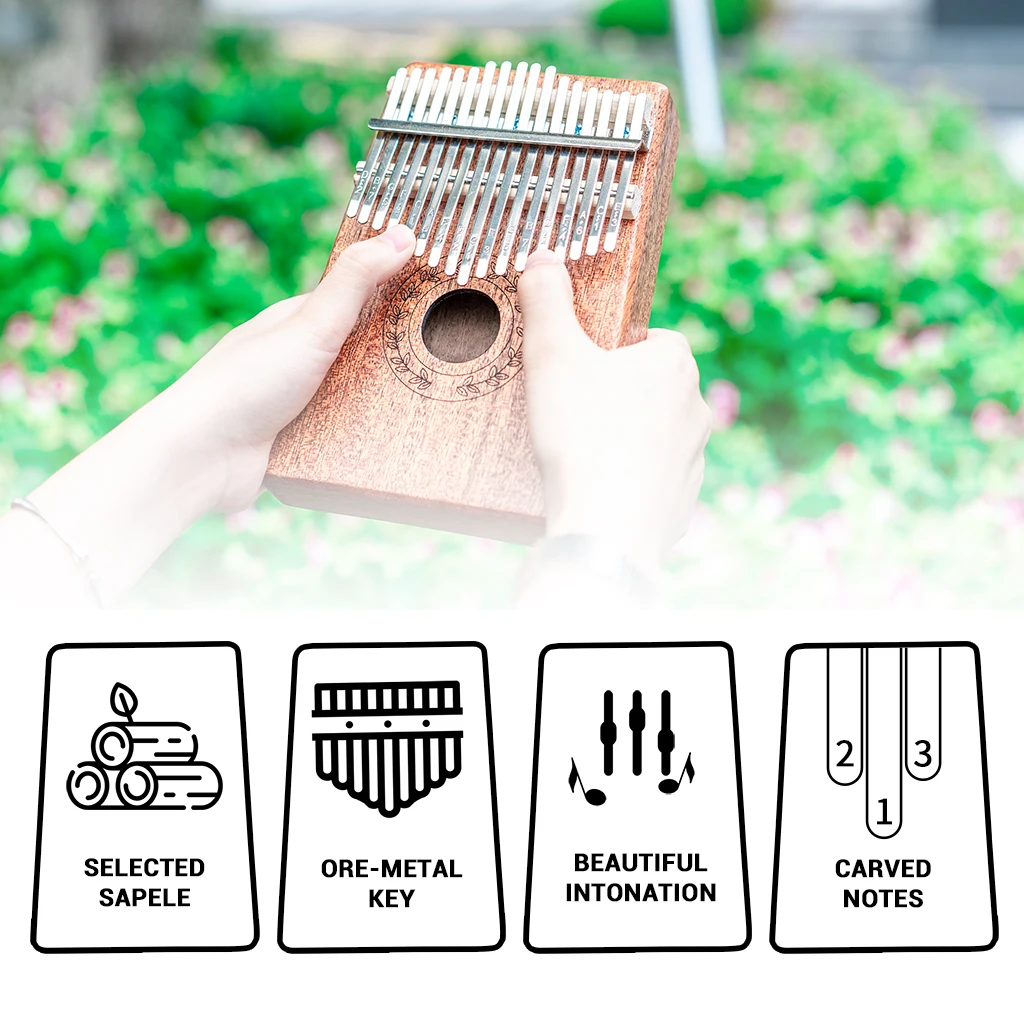The photograph showcases a wooden musical instrument, roughly rectangular in shape, held by two pale hands with thumbs poised against its metal tines for playing. The instrument features a prominent central hole adorned with concentric circles and leaf patterns outlined in black. It is set against a blurred background of lush greenery, suggesting an outdoor setting. The top part of the instrument displays around 20 metal rods of varying lengths aligned in a row, slightly spaced apart. At the bottom of the image, there are four labels with informational text about the instrument, including "selected sapele or metal key," "beautiful intonation," and "carved note." These details indicate features and characteristics, suggesting that the image serves as an advertisement for the instrument.